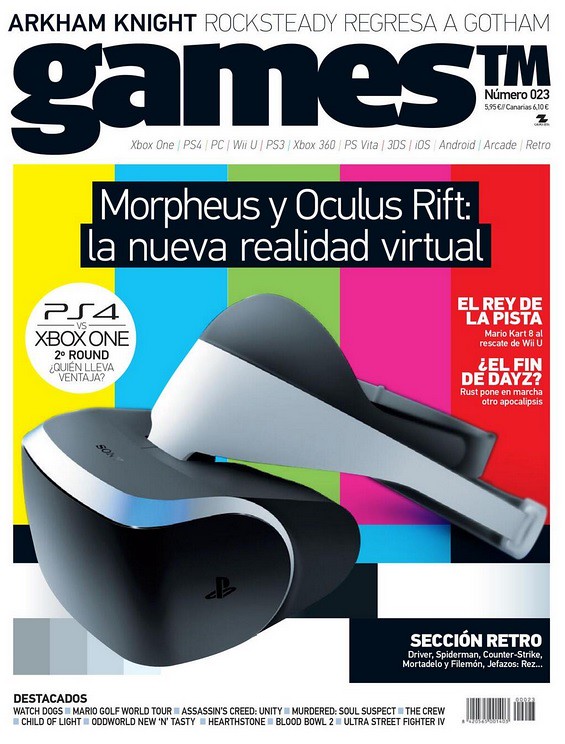This is a detailed cover photo of a tech-related magazine titled "Games TM Numero 023." At the top, it prominently features the text "Arkham Knight Rocksteady Regressa A Gotham" in large letters. Below this, there is a gray and white VR headset, identified with the text "Morpheus Oculus Rift La Nueva Realidad Virtual." The background behind the headset showcases a vibrant array of rectangular bars in yellow, blue, green, pink, and red colors, reminiscent of TV test patterns. Additional text towards the bottom lists multiple platforms including Xbox One, PS4, PC, PS3, Xbox 360, PS Vita, 3DS, iOS, Android, Arcade, and Retro, all written in black. Lastly, the bottom-right corner features barcodes. Overall, the cover incorporates a mix of English and Spanish, highlighting various gaming platforms and VR technology amidst a colorful backdrop.